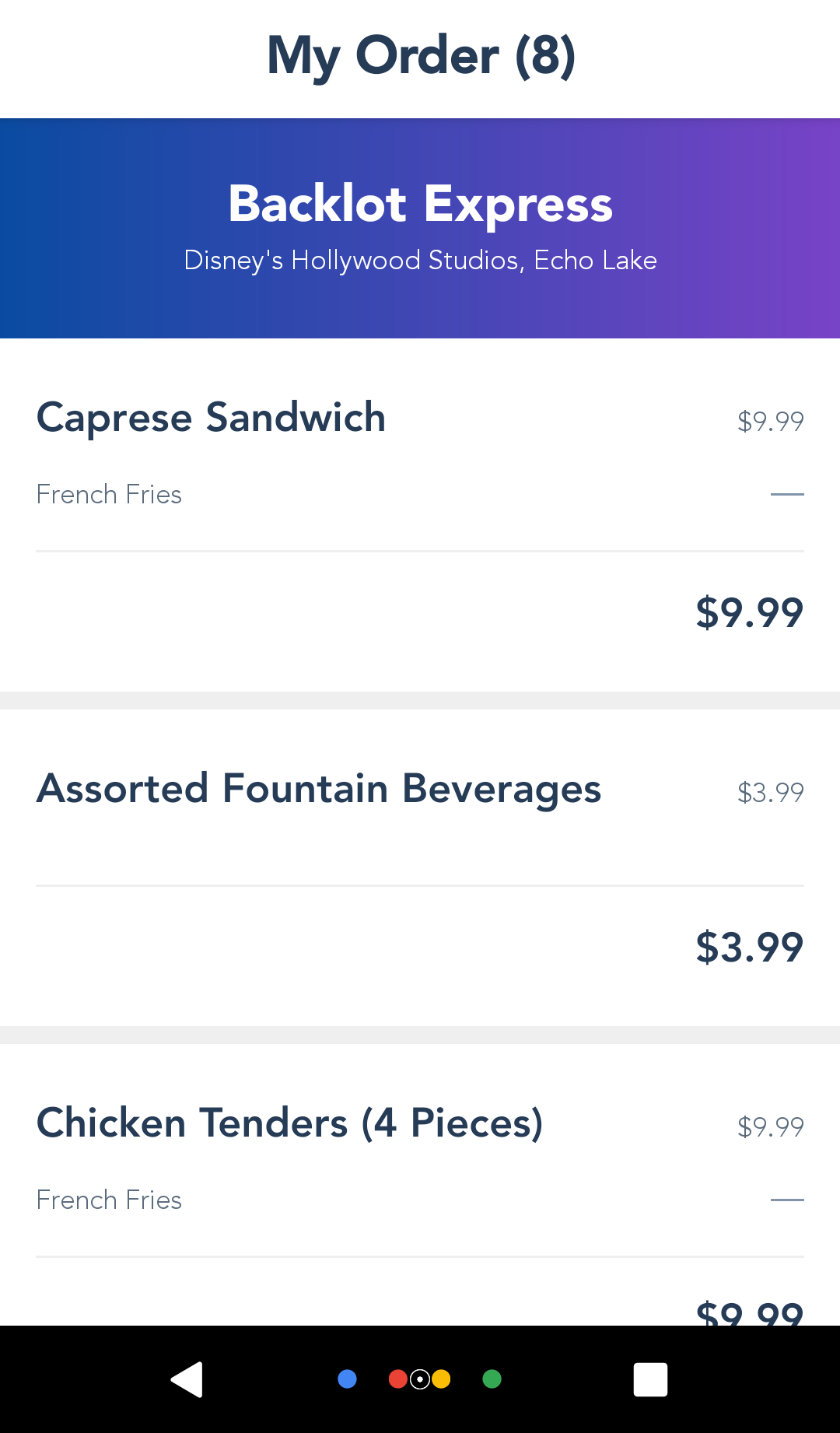A screenshot depicts a detailed order placement for the Backlot Express located at Disney's Hollywood Studios, situated in the Echo Lake area. The image is on a clean white background. At the top-center in bold black text, it reads "My Order." To the right of this header, it indicates that the order contains eight items, shown by the number "8" in parentheses. Below the header sits a gradient bar that transitions from blue on the left to purple on the right. Centered within this bar, in bold white text, is "Backlot Express," and directly beneath it, in smaller white text, is "Disney's Hollywood Studios, Echo Lake."

The order details follow below this section, presented in three distinct rows. The first item listed is a Caprese Sandwich accompanied by French fries, priced at $9.99. The second row catalogs assorted fountain beverages, each costing $3.99. Finally, the third row offers an option to choose four-piece chicken tenders served with French fries, also priced at $9.99.